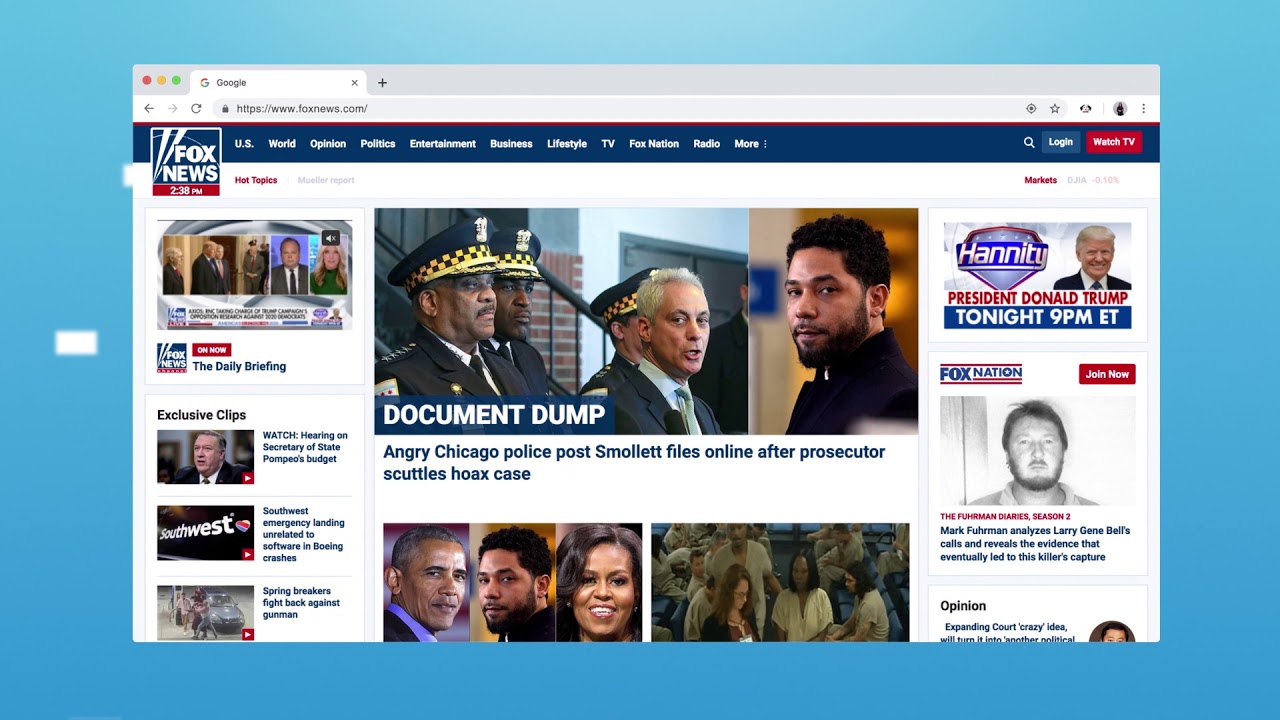This image is a screenshot of the Fox News website, captured from a laptop display at 2:38 p.m. The screenshot appears to be taken from a web browser, likely Google Chrome. 

In the upper left corner, the iconic Fox News logo is prominently displayed in its usual navy blue and red color scheme. Directly beneath the logo is the website's navigation bar, also navy blue, featuring menu options such as U.S., World, Opinion, Politics, Entertainment, Business, Lifestyle, TV, Fox Nation, Radio, and more. There's an option to log in, alongside a red text box offering the ability to watch live TV.

Dominating the central area of the screenshot is the headline for the Jussie Smollett case, captioned "Document Dump." The subtitle explains that angry Chicago police have posted Smollett files online following the prosecutor's dismissal of the hoax case. The main section includes images of police officers and Jussie Smollett.

Below this headline are three particularly notable images: portraits of Barack Obama, Jussie Smollett, and Michelle Obama, the relevance of which is not immediately clear. Adjacent to these portraits is another image, seemingly depicting nurses or attendees at a convention.

On the right-hand side of the page, there's a prominent promotion for Fox Nation, inviting users to "Join Now" and highlighting "The Furman Diaries, Season Two." 

Additionally, the main page offers exclusive clips, including coverage featuring the Secretary of State, a Southwest emergency landing involving a Boeing aircraft, and a story about spring breakers defending themselves against a gunman. A link to watch "Hannity" is also available, advertising an appearance by President Donald Trump at 9 p.m. Eastern Time.